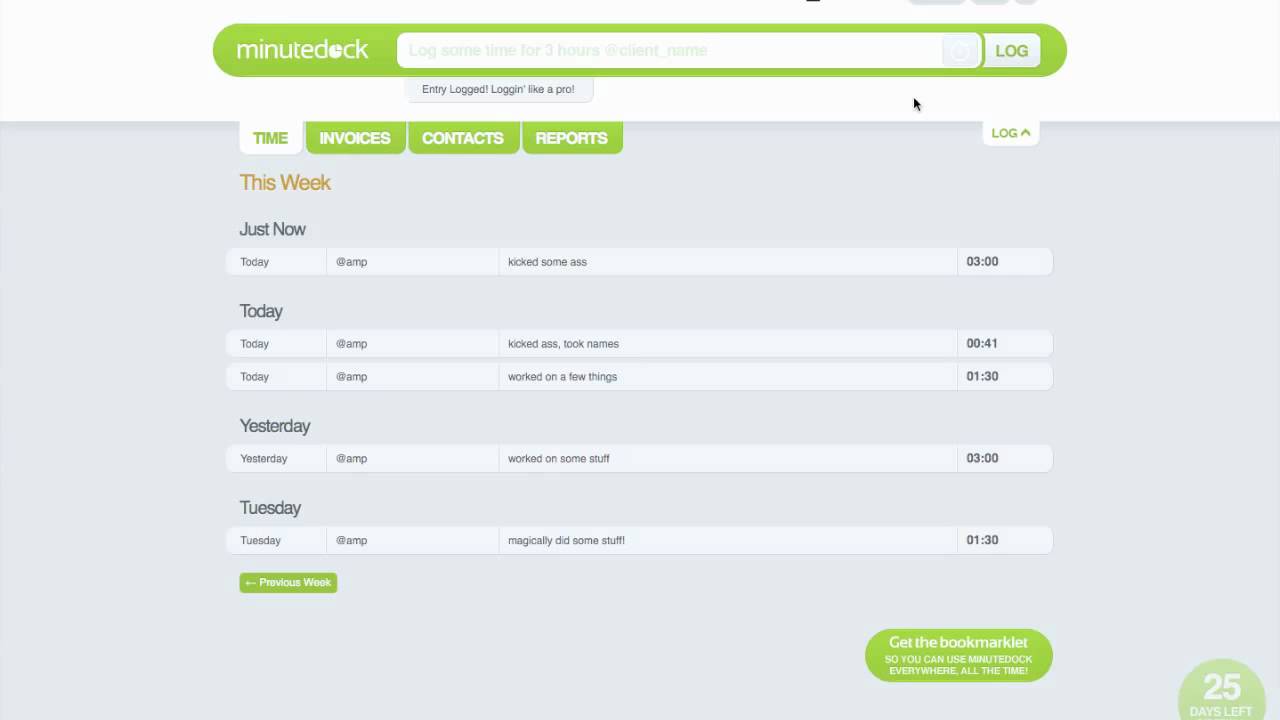The image showcases the interface of a time-tracking application named MinuteDoc. At the top of the screen, there is a long oval-shaped green banner displaying the MinuteDoc logo. Beneath this banner is a white search bar that prompts users to log time, specifically indicating "Log some time for three hours at client_name." To the right of this bar, a white button labeled "Log" is visible. 

Below the log bar, a notification reads "Entry logged" followed by the phrase "log in like a pro," complemented by a black mouse cursor icon. Directly under this, there are several tabs with the "Time" tab highlighted in white, suggesting it's the current view. The other tabs—"Invoices," "Contacts," and "Reports"—are highlighted in green.

Continuing down the interface, an orange banner displays the text "This week." Under this section, there's a chronological list of activities:

- "Just now" is followed by "Today at AMP: kick some ASS" and a timestamp of "3:00 PM."
- Below, another entry states "Today at AMP: kick ASS, took names" with a timestamp of "12:41 AM."
- Another entry indicates "Today at AMP: worked on a few things" with a timestamp of "1:30 AM."

The log then shifts to activities from the previous day labeled "Yesterday at AMP: worked on some stuff" with a time of "3:00 PM." 

Further activities are listed under specific days:
- "Tuesday at AMP: magically did some stuff" with a timestamp of "1:30 PM."

On the left side of the interface, a green button labeled "Previous Work" is visible. At the bottom right, a message encourages users to "Get the bookmark lit, so you can use MinuteDoc everywhere all the time," with a countdown indicating "25 days left."